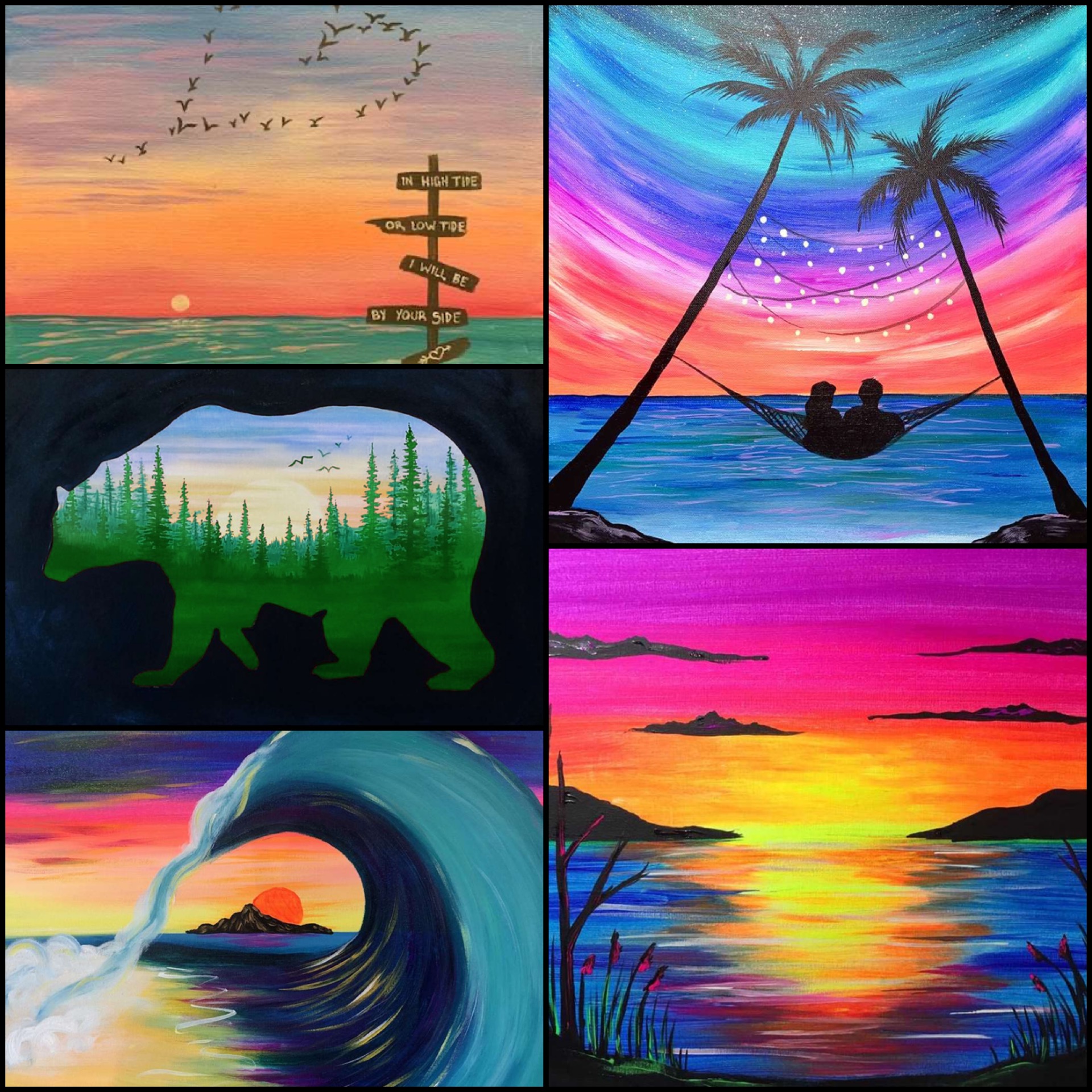This image features five distinct paintings, all rendered in a cohesive style. The top left painting depicts an ocean scene at sunset with birds flying in a heart-shaped formation against an orange sky. A series of wooden signs reads, "In high tide or low tide, I will be by your side," followed by a small heart. Below this, the middle left painting showcases the silhouette of a bear, within which a lush forest with trees, grass, and birds is intricately detailed. The bottom left painting captures a dramatic wave cresting on the water, with a black mountain and a red sun in the background. On the top right, another painting shows a tranquil coastal scene with two people lounging in a hammock strung between two palm trees, set against a vivid, colorful sky. Finally, the bottom right painting presents a serene sunset over water, featuring vibrant hues of orange, pink, and blue, with mountains and clouds in the distance.